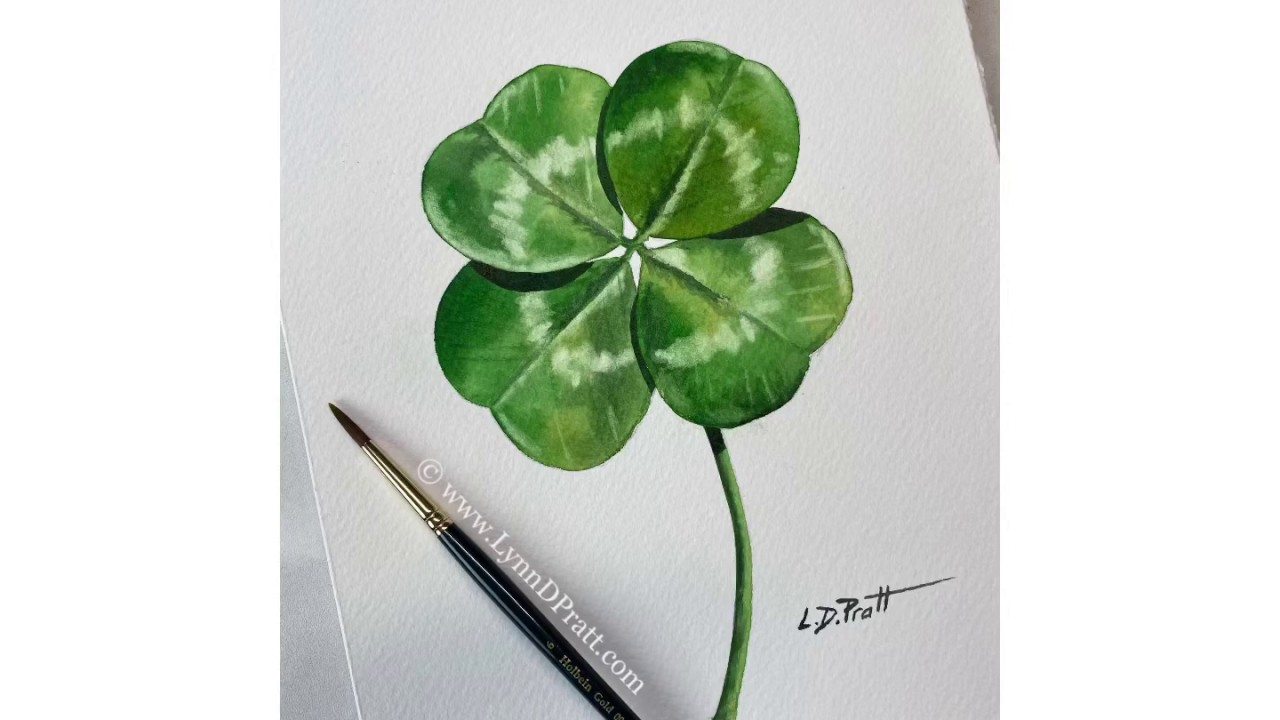The image showcases a hand-painted picture of a detailed four-leaf clover on a piece of white paper. The clover, painted in various shades of green with hints of white in the middle, features intricate vein lines on each leaf and a long stem that extends to the bottom middle of the paper. To the left of the clover, a very fine paintbrush is positioned at an angle, appearing to be staged for the photo. Above the paintbrush, the text www.lynndepratt.com is visible. The artist's signature, L.D. Pratt, is elegantly written in the bottom right-hand corner of the paper. The overall composition is simple yet striking, highlighting the detailed artwork of the four-leaf clover.